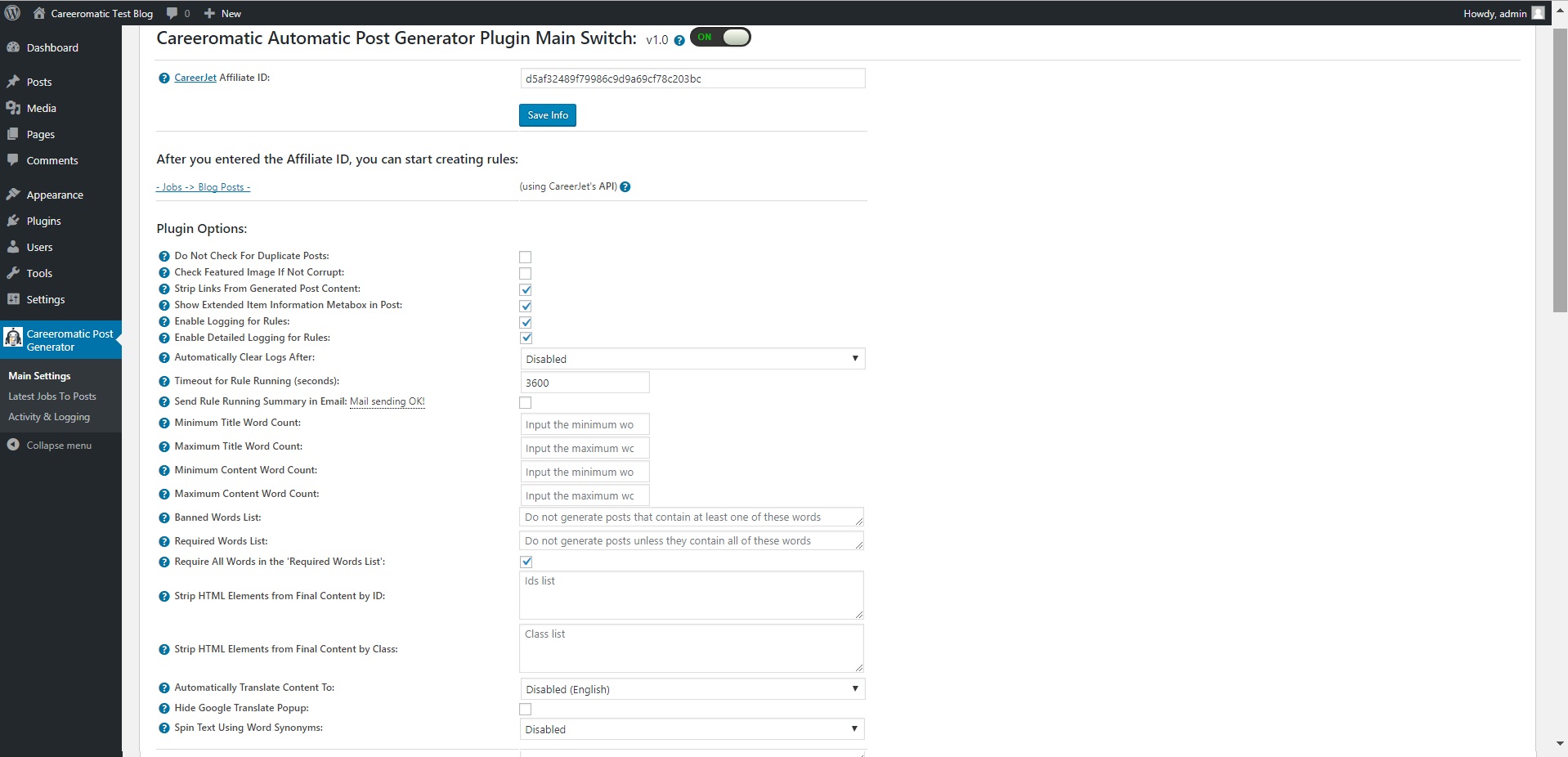This detailed image captures a zoomed-in view (at 200% magnification) of the Career-O-Matic Test Blog interface. In the upper left corner, the title "Career-O-Matic Test Blog" is prominently displayed. The left-hand side features a gray background with white text, showcasing the dashboard options such as posts, media, and pages. The currently selected option is "Career-O-Matic Post Generator," highlighted in blue. 

At the top right, there is text in white indicating "Career-O-Matic Post Generator Plug-in Main Switch," which is toggled on, signified by a green indicator and the switch being moved to the right. Below this, the affiliate ID field is filled in, accompanied by instructions that once the affiliate ID is entered, users can begin creating rules using CareerJet's API. The screen extends downward to reveal all the plugin options, which appear to be approximately 20 in total.